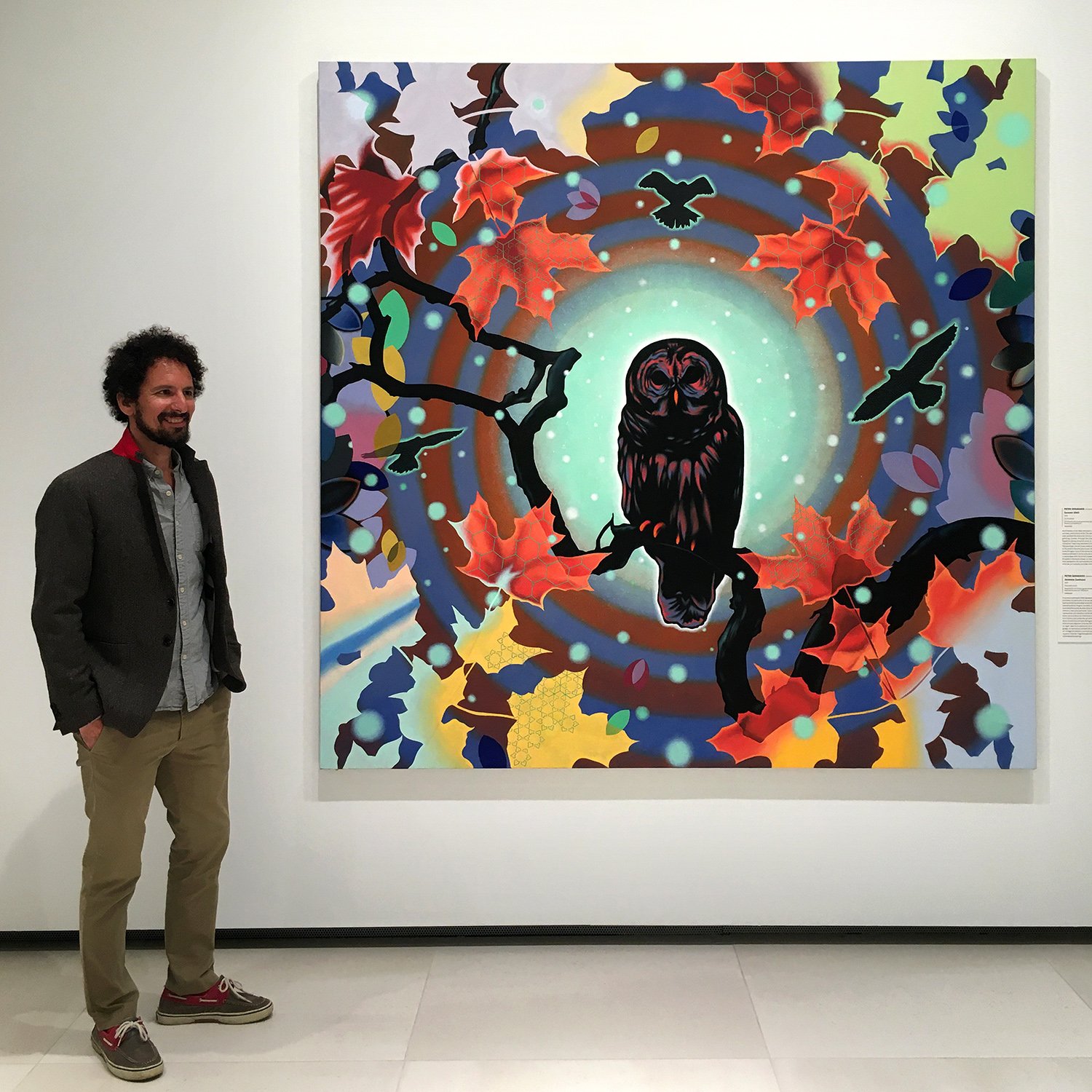This photograph captures a man standing and smiling in front of a vibrant painting hanging on a white wall. The man, likely the artist, is dressed in a gray jacket with a red collar, a gray shirt, khaki pants, and brown shoes. He has curly brown hair and a full beard. His hands are in his pockets as he looks slightly off to the right, posing confidently beside his artwork.

The painting is a captivating depiction of an owl perched on a branch at its center. The owl, rendered in black with reddish hues, is set against a dynamic background featuring swirling rings of red, blue, and yellow colors. Surrounding the owl are colorful red and blue leaves and shadowy silhouettes of other birds, which appear to be crows. The detailed artwork also includes white dots that converge into a glowing center behind the owl, enhancing the visual depth of the piece. The man’s proud demeanor and the intricate details of the painting collectively create a striking and engaging image.